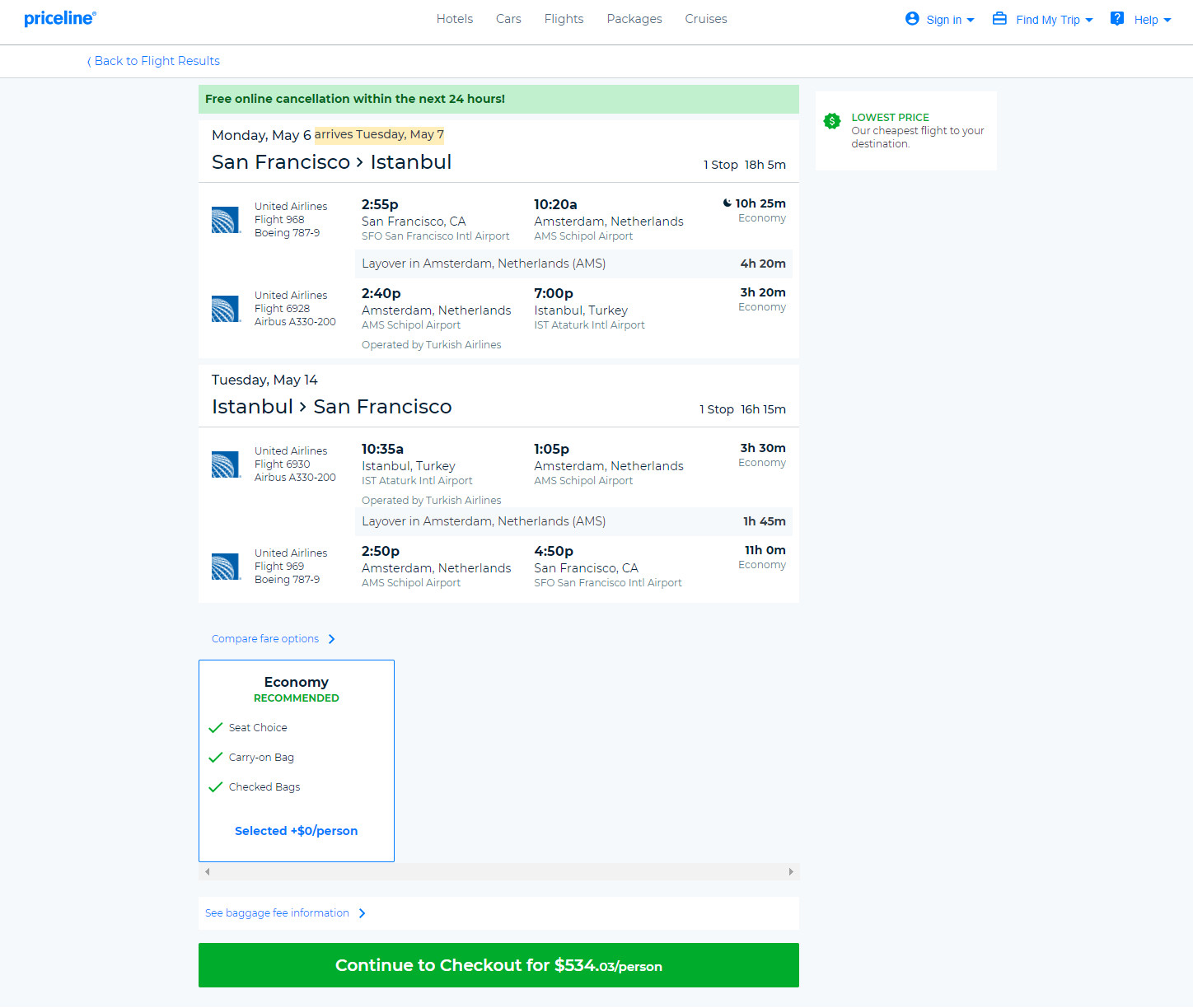This image captures the flight checkout page on Priceline. At the top, there's a header featuring the Priceline logo on the far left. Towards the center, navigation tabs allow users to access different sections of the site, including Hotels, Cars, Flights, Packages, and Cruises. On the far right, there are account settings, depicted by an icon of a person with "Sign In" text beside it, a briefcase icon with "Find My Trip" text, and a square icon with a question mark labeled "Help." 

The main content of the page focuses on booking a flight. Just below the Priceline logo on the left is a "Back to flight results" link which allows users to return to the flight selection page. Further down is a prominent green banner announcing "Free online cancellation within the next 24 hours."

Details of the booked flight are presented in two rectangular sections. The first rectangle shows a flight departing on Monday, May 6th, from San Francisco to Istanbul. It includes all relevant flight information: departure and arrival times, flight duration, economy class designation, and the number of stops.

The second rectangle contains similar information for the return flight. Beneath these sections is a categorization label for the economy class. At the very bottom of the page, a conspicuous checkout button reads "Continue to check out for $534.03 a person."